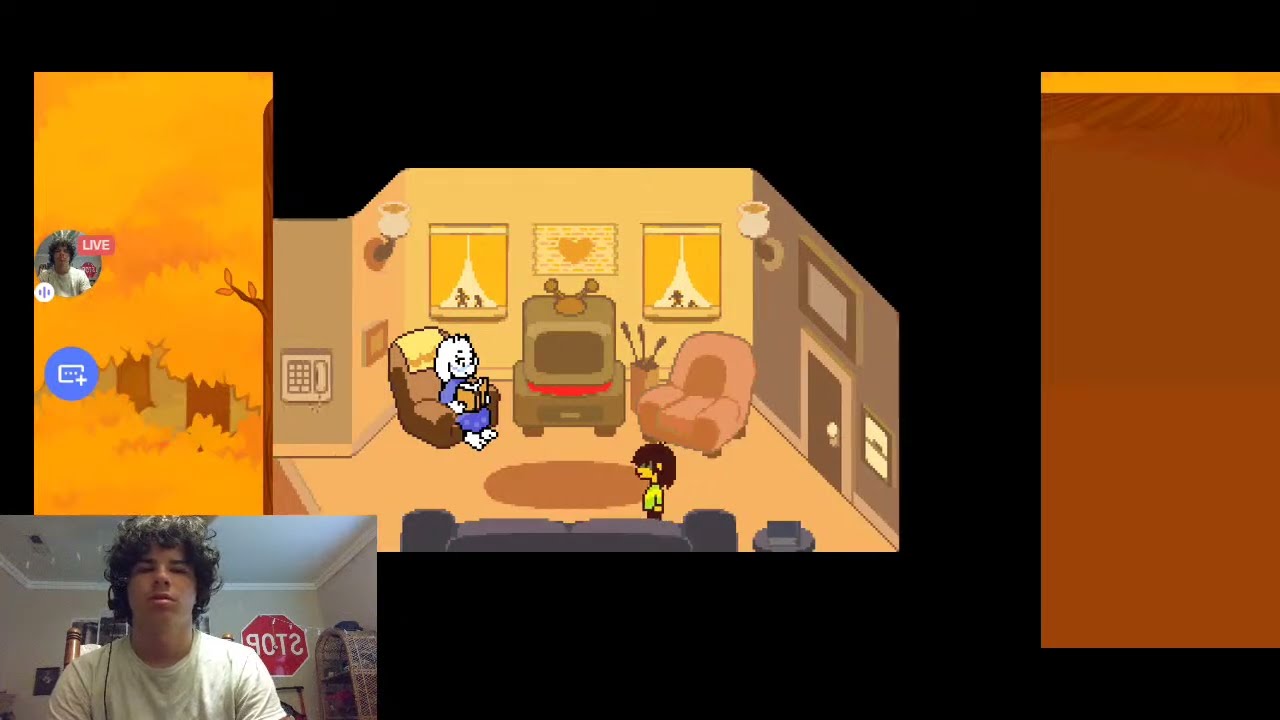The image captures a screenshot of a video game being streamed, with the streamer's webcam feed displayed in the bottom left-hand corner. The streamer, a young Caucasian male with curly brown hair, is seen in his bedroom, which features a white ceiling and a stop sign on the wall behind him. He wears a white t-shirt and is focused on the game. The streamer’s room also contains a cabinet or display unit.

The video game itself, which dominates the majority of the screen, has retro graphics reminiscent of an early or slightly improved Nintendo console. The game scene depicts a cozy living room environment. Sitting in an armchair is a white rabbit, dressed in a purple nightie, engrossed in reading a book. The living room setup includes an old-school TV, a couple of windows, a door, a wall-mounted phone, and some lamps. Another character, who appears to have dark hair and is wearing a green shirt, is present in the scene, situated near the center of the room.

Additionally, the image includes various streaming interface elements. There's a small circular icon with the streamer's picture and a rectangular widget beneath it displaying three dots and a plus sign, indicating interactive features or menu options available to viewers.